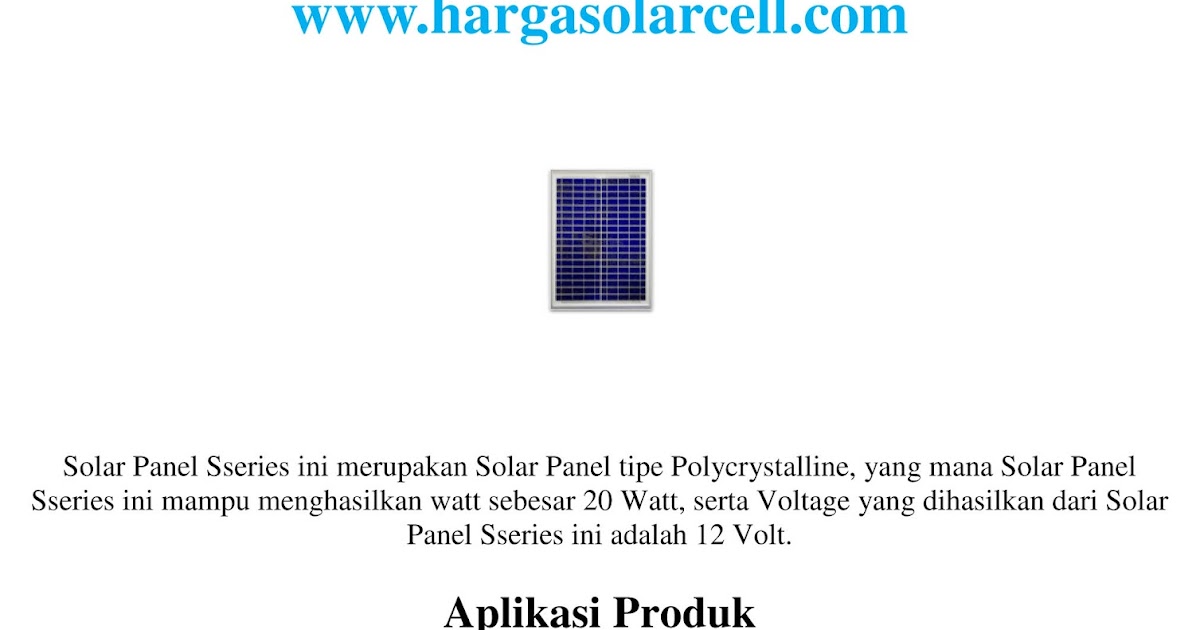The image features a small solar cell prominently centered. The solar cell has a dark indigo color with a white grid pattern. Above the solar cell, there is a bolded, blue website link in Times New Roman font that reads "www.hargasolarcell.com." Surrounding the solar cell are various texts, primarily in Arabic, discussing technical specifications related to the solar panel series, wattage, and voltage. At the bottom of the image, in bold, black Times New Roman font, there's text that reads "Aplikasa Produk," which likely indicates a product label from a company possibly named Aplikasa. The overall background of the image is white, creating a clean and clear advertisement layout for the solar cell company.